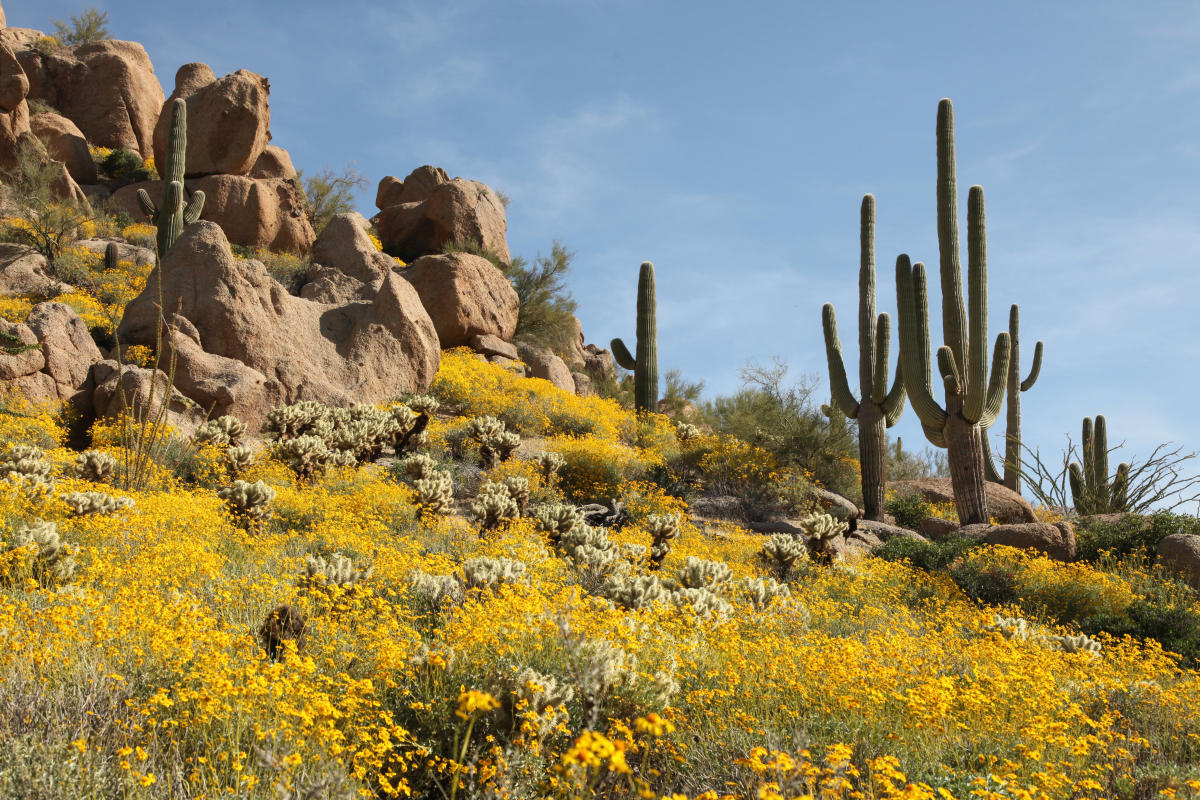A daytime photograph, likely taken in the American West or Midwest, depicts a semi-arid landscape characterized by iconic large cacti reminiscent of those often seen in cowboy movies. The scene features a mix of sandy and grassy terrain with patches of greenery, suggesting a climate that fluctuates between dry and slightly more verdant periods throughout the year. The ground is adorned with numerous yellow and white flowers, potentially allergenic for some, and dotted with sparse grass or weeds. Prominent in the foreground and to the right are several towering cacti, about four to six in number, with some additionally protruding from behind a cluster of sizable, easily dislodged boulders. The backdrop showcases a wide expanse of clear blue sky, accented by a few wispy white clouds, adding to the serene yet warm atmosphere of the image.